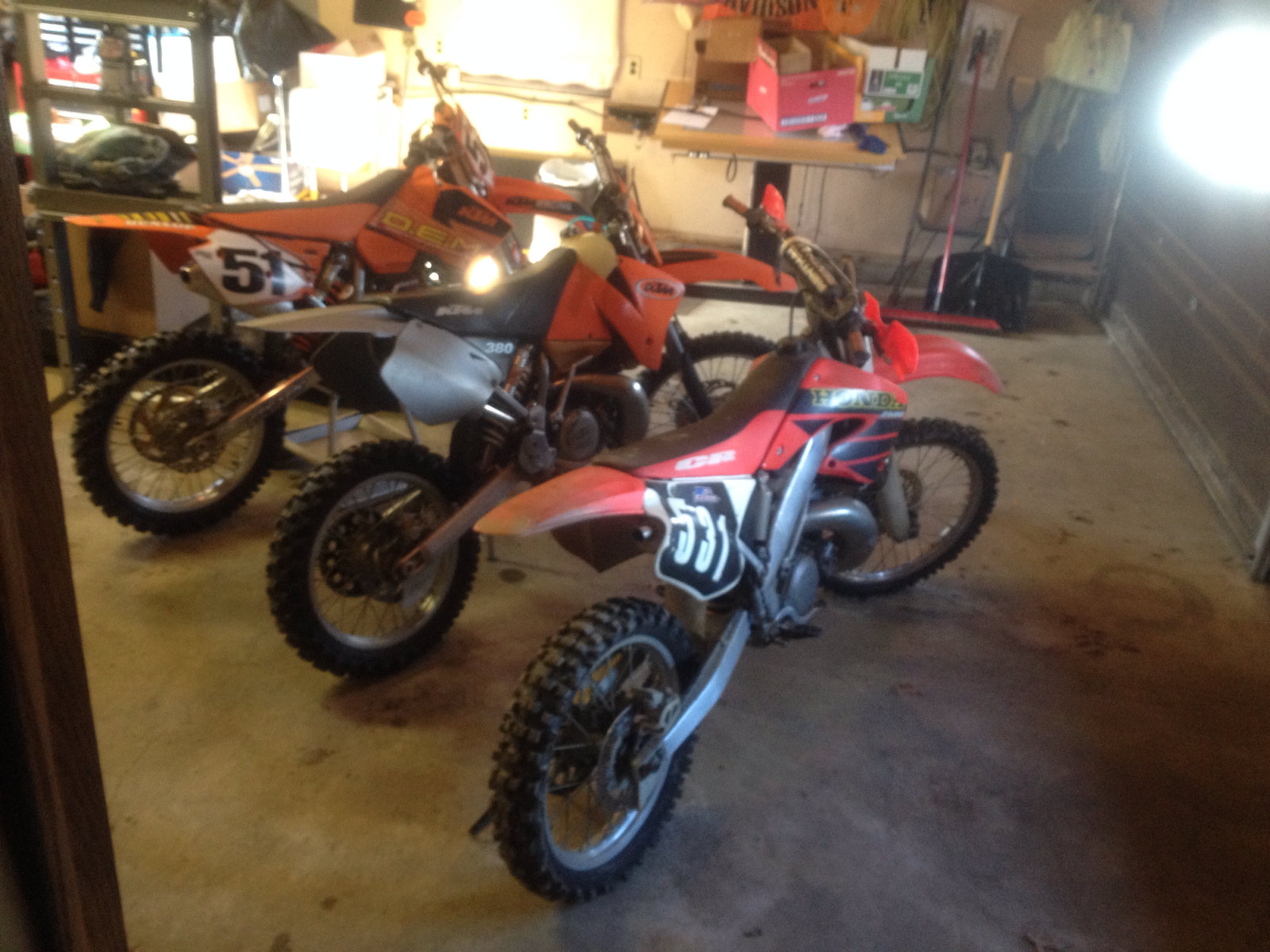The detailed image depicts a cluttered home garage with a stained, light-colored cement floor. Three red and black dirt bikes, all facing the right-hand side of the picture, are the central focus. The bike closest to the foreground features the number 531 and bears the brand name "Honda," while the bike furthest back displays the number 51 (or possibly 5051) and another bike has a visible number 380. The garage's back wall is lined with shelves holding various items, including snow shovels, tools, and red boxes. A window at the top center of the image allows sunlight to stream in, casting light on the scene. Additionally, metal racks and more tools are visible on the top left side. The garage door is on the right, partially allowing light to spill in, adding a white glow to that side of the image. The dirt bikes have knobby tires and black handlebars, hinting at a dirt bike racing hobby.